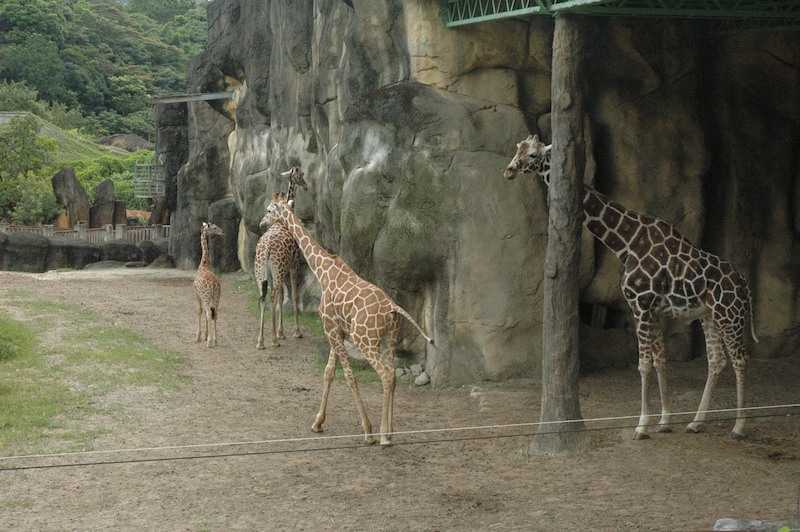This exterior shot, taken from a visitor's perspective at a zoo, captures a detailed scene of a giraffe enclosure. The top left of the image reveals a dense mass of trees and hills, gradually giving way to smaller trees, shrubs, and scattered rocks. A fence runs around this area, enhancing the zoo-like setting. The main focal point is a large, multi-colored rock formation with shades of gray, green, light tan, and white spots, dominating the top and right-hand side of the image. The ground is mostly barren with patches of grass and dirt, particularly noticeable in the right-hand side and bottom sections.

Four giraffes are depicted within this enclosure. Their coats display the characteristic brown, towel-like patches separated by thin tan lines. Notably, one giraffe appears significantly smaller, likely a baby, standing near the back with another giraffe, both facing the rock formation. The central giraffe also looks towards the back, while the fourth and largest giraffe stands under a cover on the right side, darker in color compared to its companions. Additionally, two black and white containment wires run across the bottom of the image, with a wooden tree post supporting a green railing visible in the top-right section.